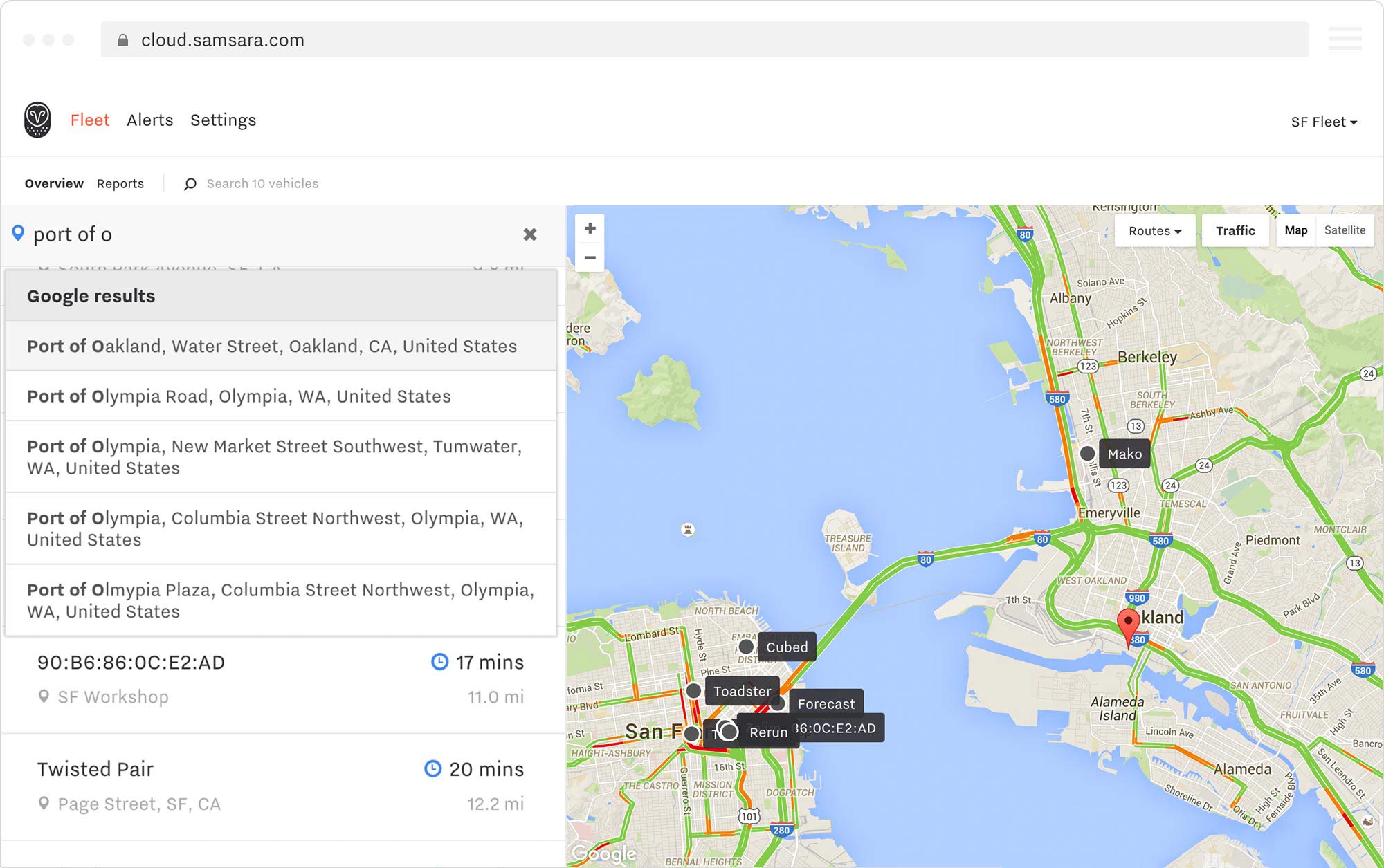The image is a screenshot, likely from a desktop or laptop, with dimensions fitting a long rectangle, which is wider than it is tall. The main application shown is Google Maps, although the focus is on a different interface overlay. The URL at the top reads "cloud.samsara.com". Beneath the URL bar, there are three prominent tabs labeled "Fleet", "Alerts", and "Settings". The "Fleet" tab is currently selected, indicated by its orange text, in contrast to the black text of the other tabs.

Directly below these tabs, the word "Overview" is highlighted, showing it is the current sub-section in use. In the main part of the screen, there is a list labeled "Google results," which includes various locations such as "Port of Oakland, Water Street, Oakland, California", and several locations in the Port of Olympia area including "Port of Olympia Road", "Port of Olympia, New Market Street", "Port of Olympia, Columbia Street", and "Port of Olympia Plaza, Columbia Street Northwest".

To the right, a section of Google Maps displays an overhead view of Oakland and San Francisco, highlighting the waterway and the bridge that connects these two cities. A location pin is visible in Oakland, accompanied by several floating gray text boxes labeling different locations with names like "Mako", "Cubed", and "Toadster". The exact nature of these names is unclear, but they appear to denote specific locations on the map.